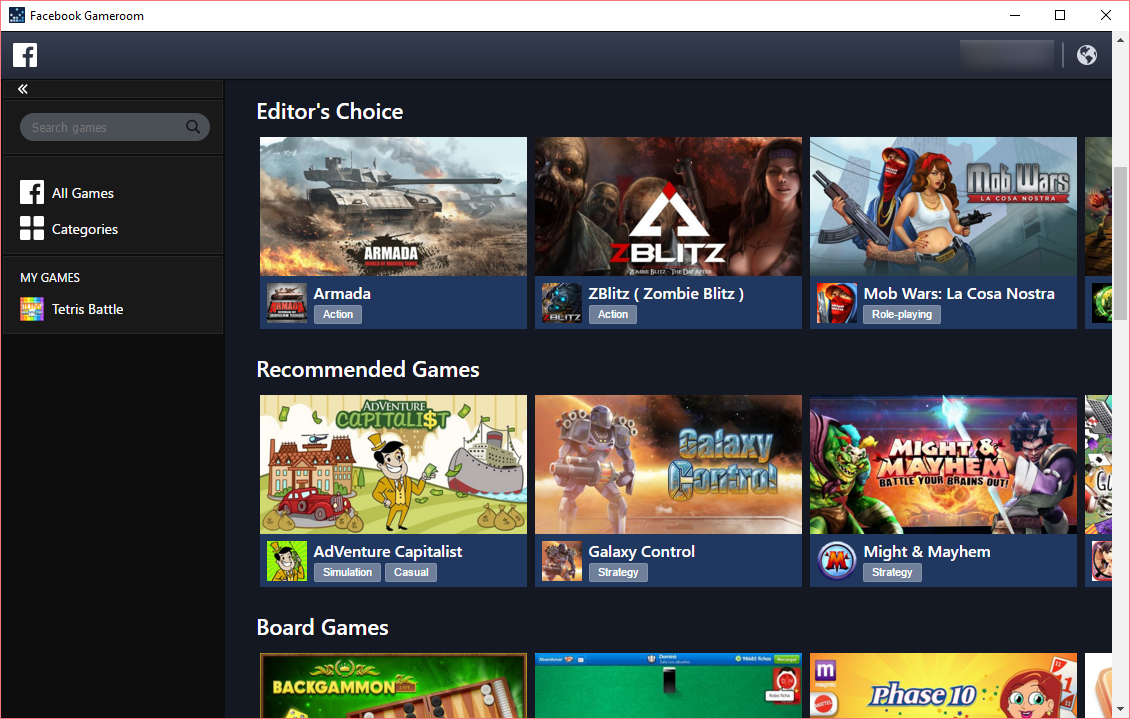This image is a screenshot of the Facebook Game Room interface, showcasing a well-organized and visually appealing layout designed for easy navigation. At the top, the title "Facebook Game Room" prominently signals the application in use. The left sidebar features various categories, including "Search Games," "All Games," "Categories," and "My Games," with "My Games" specifically highlighting "Tetris Battle."

The main interface is divided into several sections featuring a variety of game recommendations. The "Editor's Choice" category displays "Armada," "Z Blitz" (an action-packed zombie game), and "Mob Wars: La Cosa Nostra," a role-playing game with a dramatic cover image of characters clutching weapons in an urban setting.

In the "Recommended Games" section, "Adventure Capitalist," a simulation and casual game, is shown with a cartoon-style cover image of a man in a suit reminiscent of the Monopoly man. Other recommended games include "Galaxy Control," a strategy game with a futuristic theme featuring a soldier or robot on the cover, and "Might and Mayhem," another strategy game with animated, vibrant characters engaged in battle.

A cut-off portion of the "Board Games" section reveals titles like "Backgammon Live," a classic board game, "8 Ball Pool," and "Phase 10," a card game. The layout is meticulously designed to be both intuitive and visually appealing, enriched with high-quality images and clear labels for all the games, making it user-friendly and engaging for players of all interests.